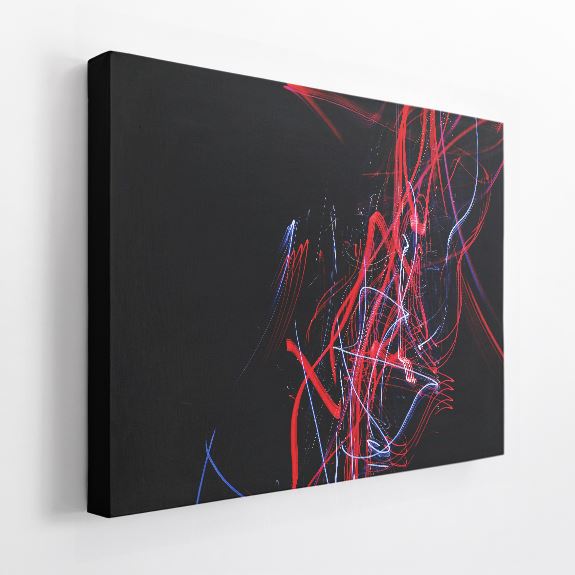This photograph captures a large, rectangular canvas mounted on a clean, white wall. The piece, which resembles a painted acoustic panel, is a striking example of abstract modern art. With a predominantly black background, the artwork features vivid, squiggly lines and swirling patterns in red, blue, and white. Most of these colorful elements are concentrated on the right side of the canvas, some trailing vertically with others veering horizontally. The left side of the panel is mostly black, creating a stark contrast and drawing attention to the dynamic lines on the right. The image is taken in a square format with the canvas hung in a landscape orientation, and there’s a light source illuminating the right side, adding a subtle glow to the vibrant colors. The minimalistic white wall serves as a perfect backdrop, enhancing the overall impact of this impressive piece of artwork.